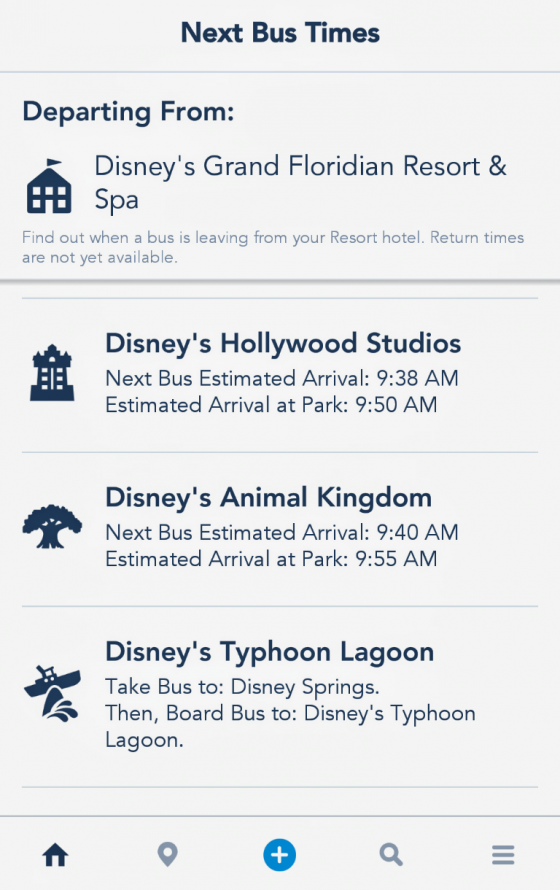The image is a screenshot displaying bus schedules on a light gray background with black text. At the top center, bold black text reads, "Next Bus Times," with a horizontal light gray line running beneath it. Below this line, the text indicates departure information: "Departing from Disney's Grand Floridian Resort and Spa. Find out when a bus is leaving from your resort hotel. Return times are not yet available."

Following this, the destinations are organized in sections:

1. **Disney's Hollywood Studios**: 
   - The title is presented in bold black text.
   - Information beneath: "Next bus estimated arrival: 9:38 a.m. Estimated arrival at park: 9:50 a.m."
   
2. **Disney's Animal Kingdom**: 
   - Alongside the destination title, there's an illustrated black tree to the left.
   - Information beneath: "Next bus estimated arrival: 9:40 a.m. Estimated arrival at park: 9:55 a.m."

3. **Disney's Typhoon Lagoon**: 
   - Instructions for reaching the destination: "Take bus to Disney Springs then board bus to Disney's Typhoon Lagoon."

Each segment clearly indicates the estimated arrival times for the next buses and provides specific details for guests departing from Disney's Grand Floridian Resort and Spa.